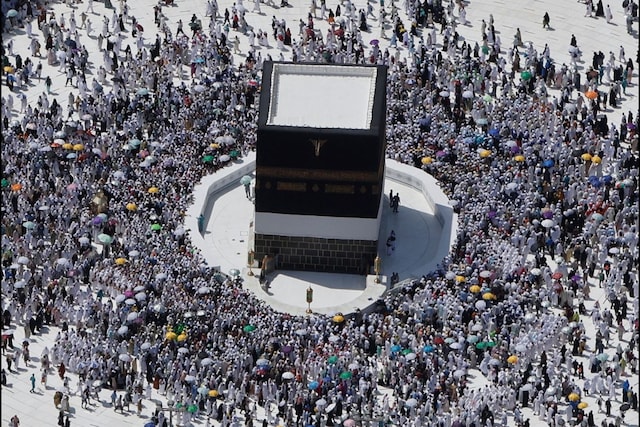The image is a high-angle photograph depicting the religious ritual of Tawaf in Mecca, a central pilgrimage in the Muslim faith. At the heart of the image stands the Kaaba, a tall and predominantly black cubic structure, adorned with a band of white and a gold trim near its top, and capped with a white or cream-colored roof. The Kaaba is surrounded by a clear, circular area that separates it from the dense crowd of pilgrims. The crowd, which appears as a mass of small, blurred dots from this aerial perspective, predominantly wears white and gray, traditional attire. Scattered among the pilgrims are various colored umbrellas providing shade, adding splashes of yellow, green, blue, and orange to the scene. The photograph captures the essence of this significant Islamic ritual, emphasizing the unity and devotion displayed by the gathered worshipers.